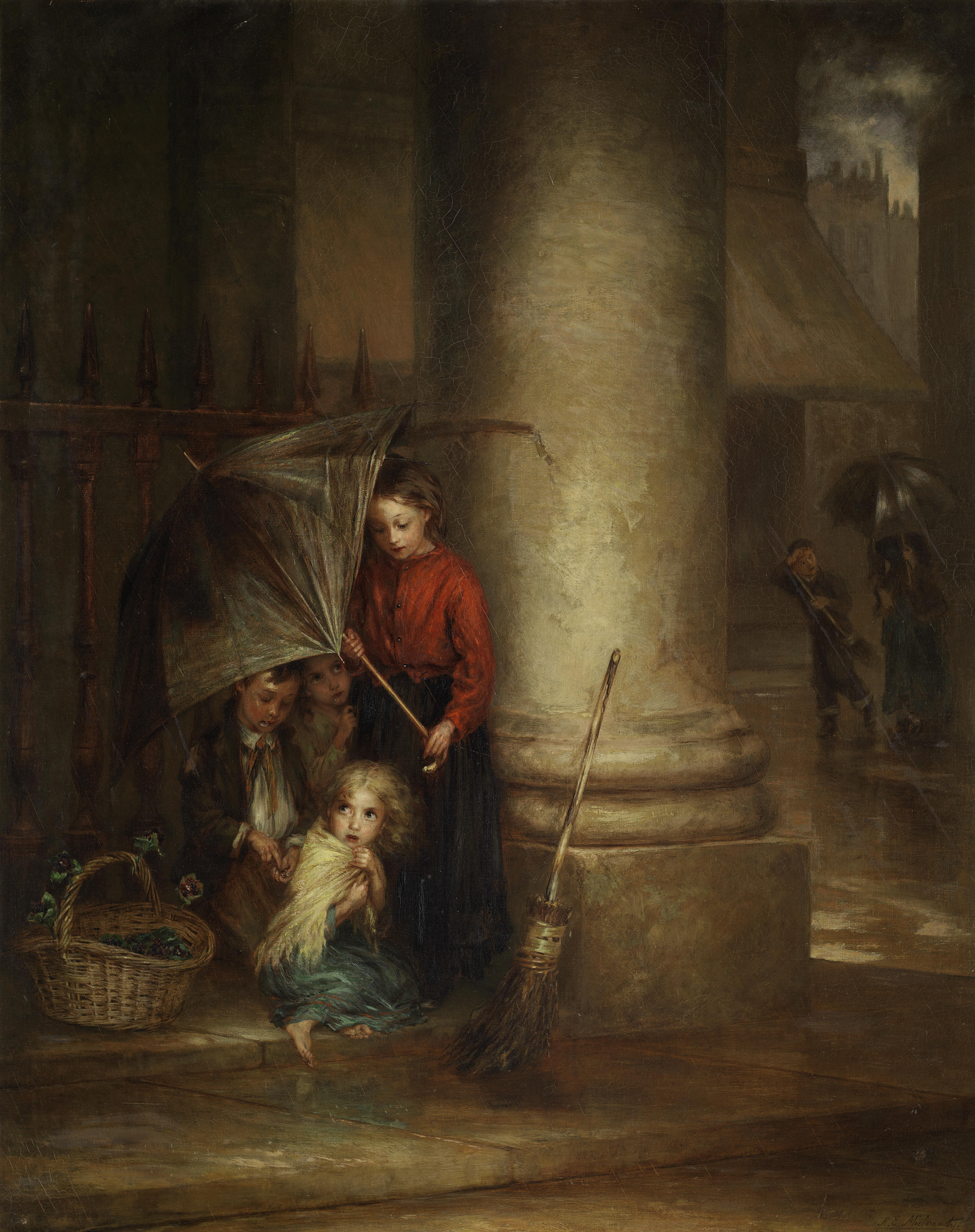The painting depicts a dark, gloomy street scene under a rainy sky, with thin white streaks representing the falling rain. Dominating the center of the image is a large white stone column, against which an old-fashioned straw broom is leaning. At the base of the column, a young girl wearing a red, long-sleeved blouse and a long black skirt holds a dilapidated black umbrella, sheltering three other children. 

To her right is a girl clutching her skirt, while a boy in tattered clothes with an downcast gaze stands next to her. Another young girl, barefoot with blonde hair, wearing a white shawl and blue dress, is positioned at the front. Beside them, there is a picnic basket on the ground.

In the background, dark tan or brown buildings contribute to the somber mood, and two more individuals, a man and a woman, are partially visible to the right, also holding an umbrella. The far distance reveals the faint, blurry outline of a castle, adding to the atmospheric setting. The entire scene is framed by the presence of a wrought iron fence, enhancing the feeling of an old, rain-drenched, urban environment.